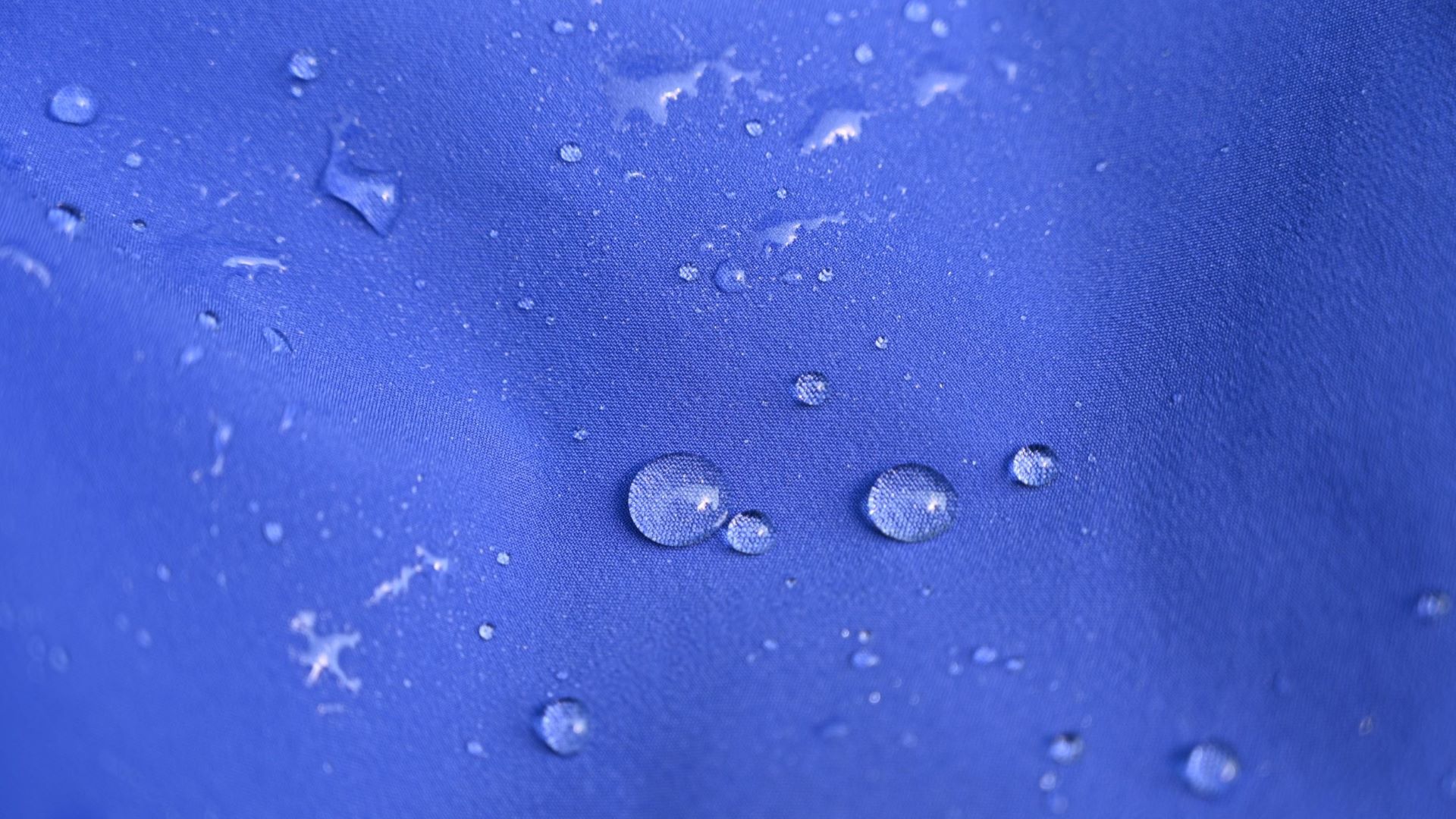This color photograph, in a landscape orientation, showcases a blue woven fabric or cloth, featuring a series of water droplets scattered across its surface. The fabric, which may be treated with a water-repellent coating, appears primarily medium blue with slight variations and ripples that produce highlights and lowlights. The water droplets exhibit various forms, from perfectly formed elliptical shapes in the center to smeared and flatter droplets towards the top, and numerous smaller, circular beads dispersed randomly. The droplets magnify the intricate texture of the cloth, revealing fine, barely visible weaves and small bumps. The overall scene suggests a material that exhibits water resistance, similar to a raincoat or a highly absorbent cloth like a shamwow. The light source and the setting, whether indoors or outdoors, remain ambiguous, but the image captures the realistic and detailed interaction between water and the textured fabric.